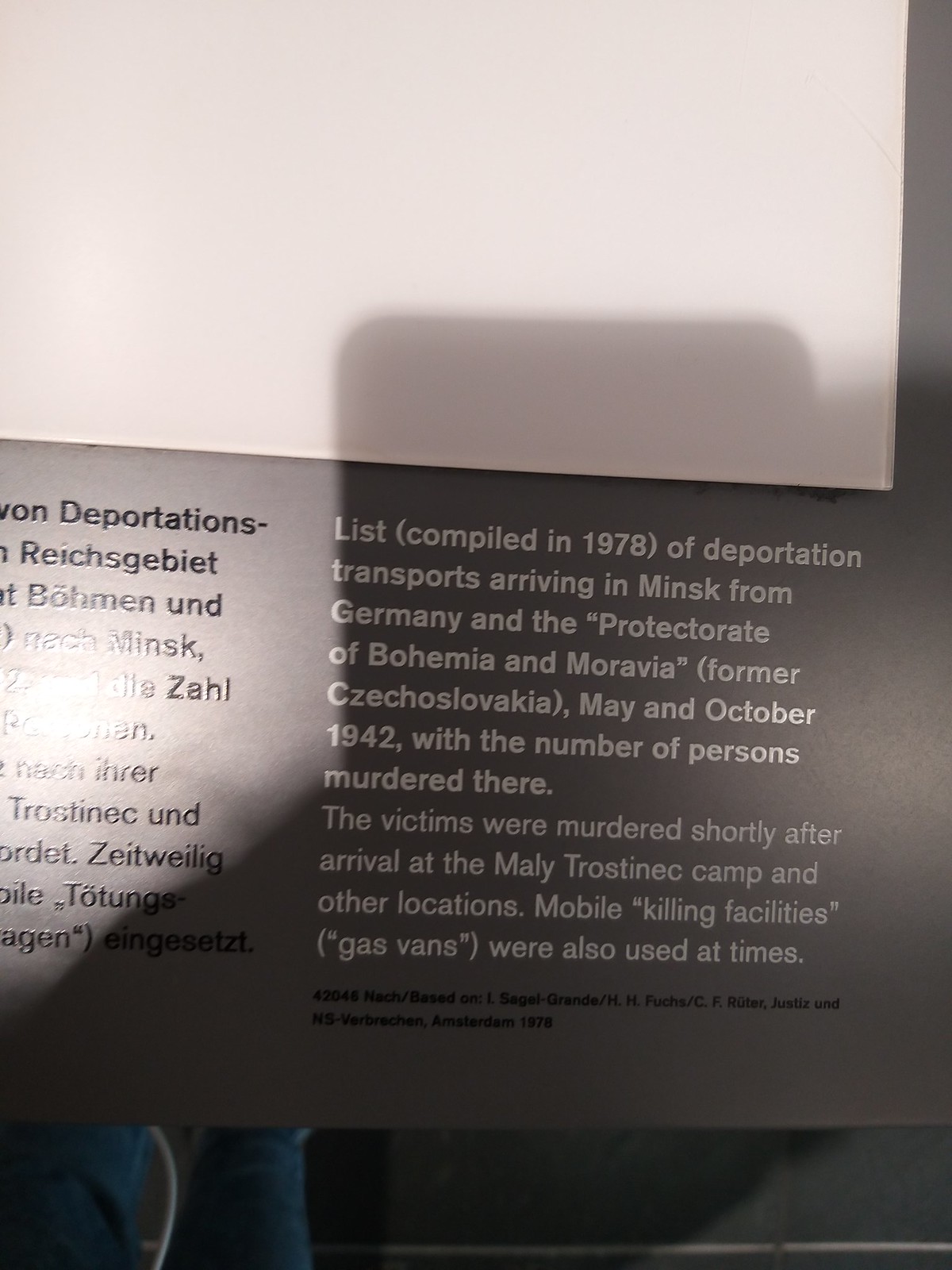This photograph likely taken in a museum or historical exhibit, showcases part of a poster or display detailing a tragic period from World War II. In the top-right corner, a white section is visible, and beneath it, against a gray background, there are two columns of text. The left column, partially visible, appears to be in German, while the right column is in white font. It states: "List compiled in 1978 of deportation transports arriving in Minsk from Germany and the Protectorate of Bohemia and Moravia, May and October 1942, with the number of persons murdered there." It goes on to explain that upon arrival at the Maly Trostenets camp and other locations, many victims were murdered shortly thereafter, often utilizing mobile killing facilities such as gas vans. This somber piece likely serves to educate visitors about the horrors faced by deportation victims during the Holocaust.